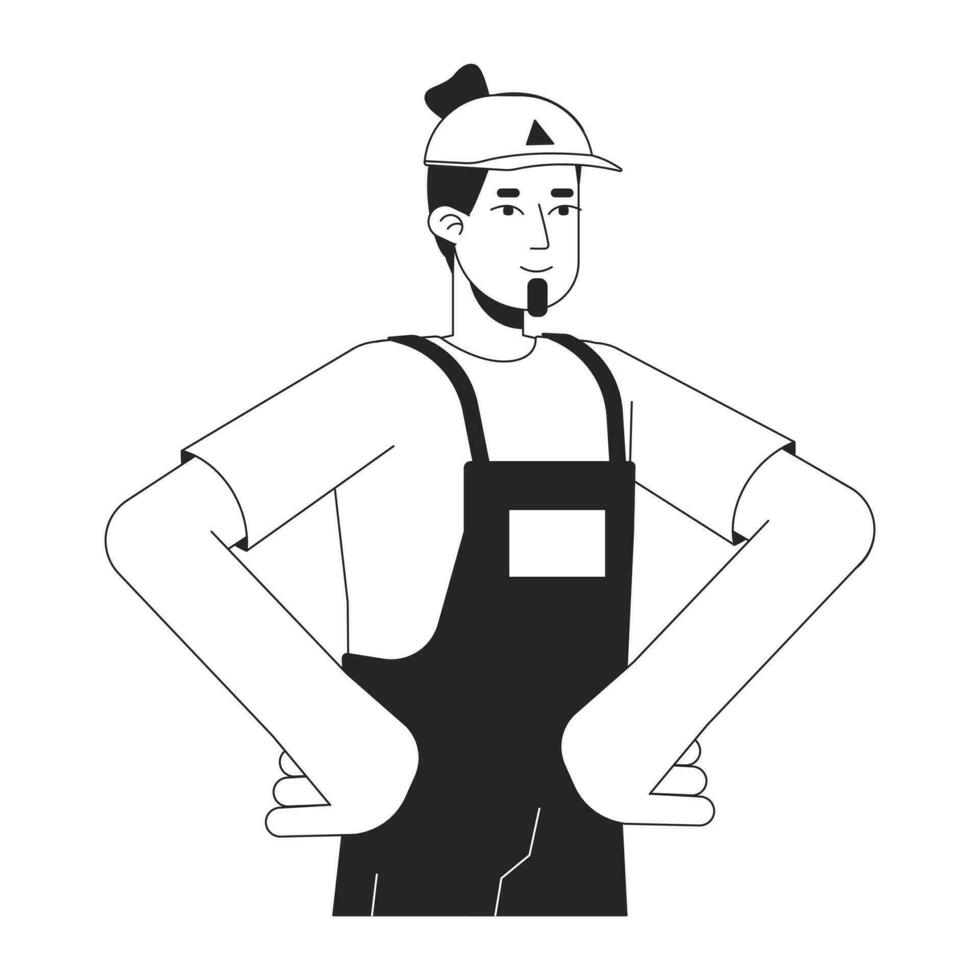This stock illustration, set against a stark white background, depicts a cartoonish man in a service uniform. The character is dressed in a black apron with no writing on it, over a white short-sleeved t-shirt, and wears a baseball cap adorned with a black triangle logo. The man's hair is tied up into a small man bun peeking from the back of his cap, and he has a black goatee. His exaggeratedly wide arms rest on his hips, forming pronounced triangular shapes against his sides. The image, entirely in black and white, captures a relaxed, smiling expression, accentuated by stylized eyebrows and a forward-looking gaze. The highly stylized, disproportionate forearms and minimalistic color scheme suggest it is commonly used for advertisement purposes.